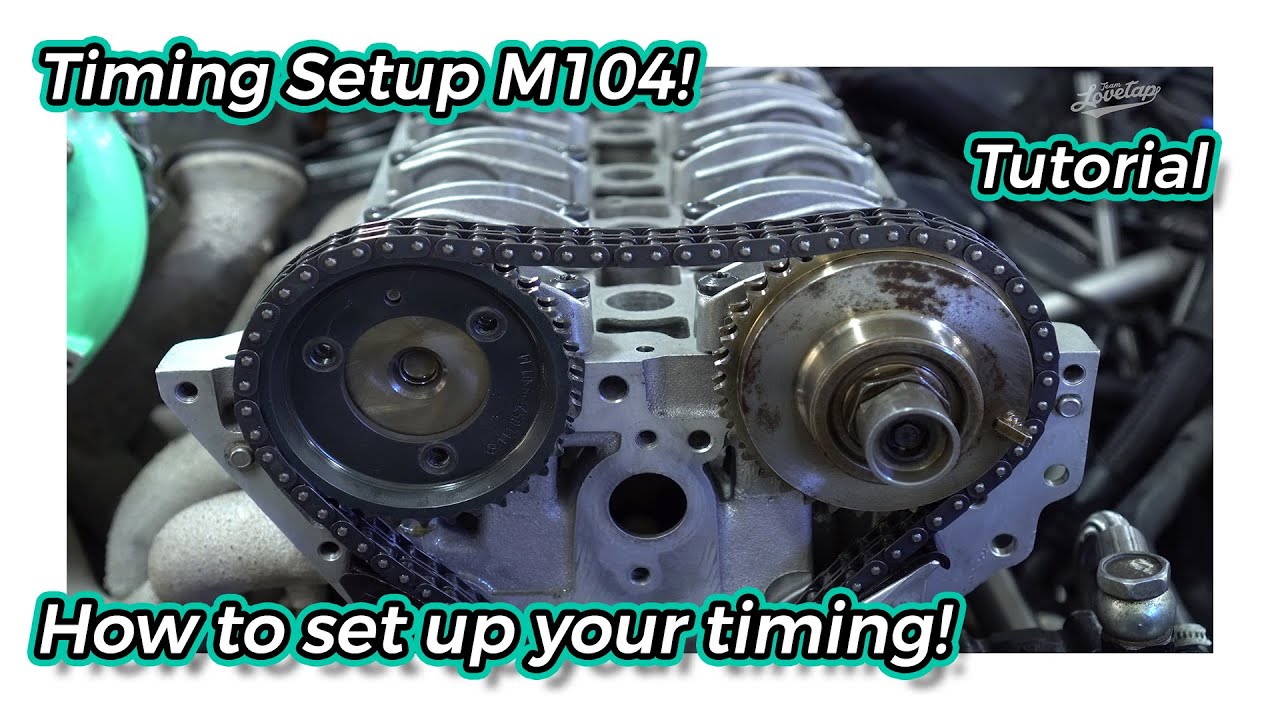The image depicts a detailed view of an engine setup, likely an eight-cylinder configuration with a chain drive mechanism. At the front, two large metal gears are interconnected by a chain, resembling a bike chain, which extends downward to a less visible gear. Surrounding the well-lit machinery are various mechanical parts, with a teal-colored component on the left, possibly a coolant reservoir. The image is part of a tutorial, as indicated by the white text with black and teal borders: "Timing Setup M104!" in the top left corner, "Tutorial" and "Love Tap" on the top right, and "How to set up your timing!" in the bottom left. The background is intentionally blurred to emphasize the engine, making the textual guidance the only other clear element in the image.